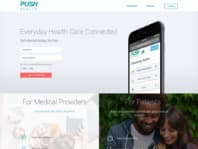The image features a mobile device displaying a somewhat blurry page, where a sign-up or sign-in field is noticeable. Towards the bottom of the image, there is a happy couple—a man and a woman—who are looking down at something, smiling. Behind them, a vibrant garden wall adorned with lush green grass creates a serene backdrop. The text on the page includes a mix of blue, orange, and grey colors, contrasting against black and white elements. No additional details are present in the image.